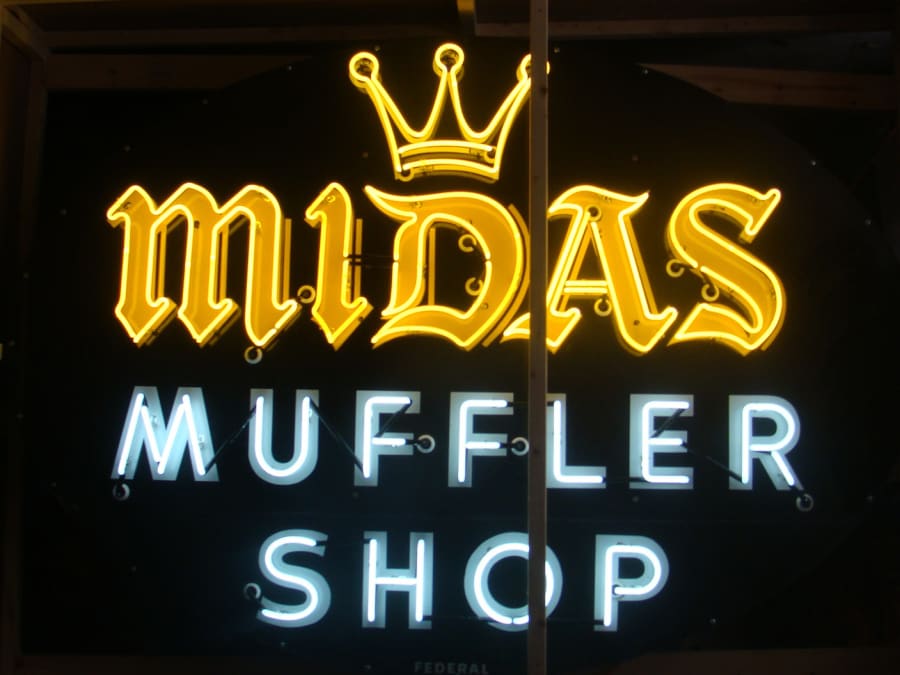The image showcases a neon sign for the "Midas Muffler Shop" glowing brightly against a dark, nighttime background. The top part of the sign displays the word "Midas" in a golden, almost old-timey font, highlighted by a three-pointed crown also in gold neon above the "D". Below "Midas," the words "Muffler Shop" are illuminated in light blue neon, presented in plain block letters. A metal pole runs vertically through the image, slightly to the right of center, partially obscuring some of the letters. The background is predominantly black, with some visible fixtures and light bulbs hinting at the structure supporting the sign. The overall effect is a vivid contrast of yellow and blue neon lights against the dark surroundings.